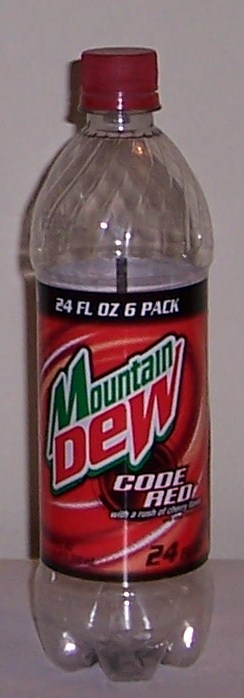This is a detailed picture of an empty Mountain Dew Code Red bottle. The clear plastic bottle, distinguished by its red cap with an unbroken red seal ring, rests against a white wall atop a white platform. Illuminated by a frontal light, the bottle casts a pronounced shadow behind it. The label is predominantly red with intricate white and black swirls, and it features a striking design with “Mountain Dew” prominently displayed—the word "Mountain" in green and "Dew" in red. The "Code Red" insignia is presented in bold white text outlined in black, located at the bottom right beneath the "W" of "Dew." Notably, the label's black upper border contains the text “24FLOZ6PK” in white, indicating the bottle originally came from a six-pack collection. The capacity, "24 oz," is specified at the bottom right of the label.